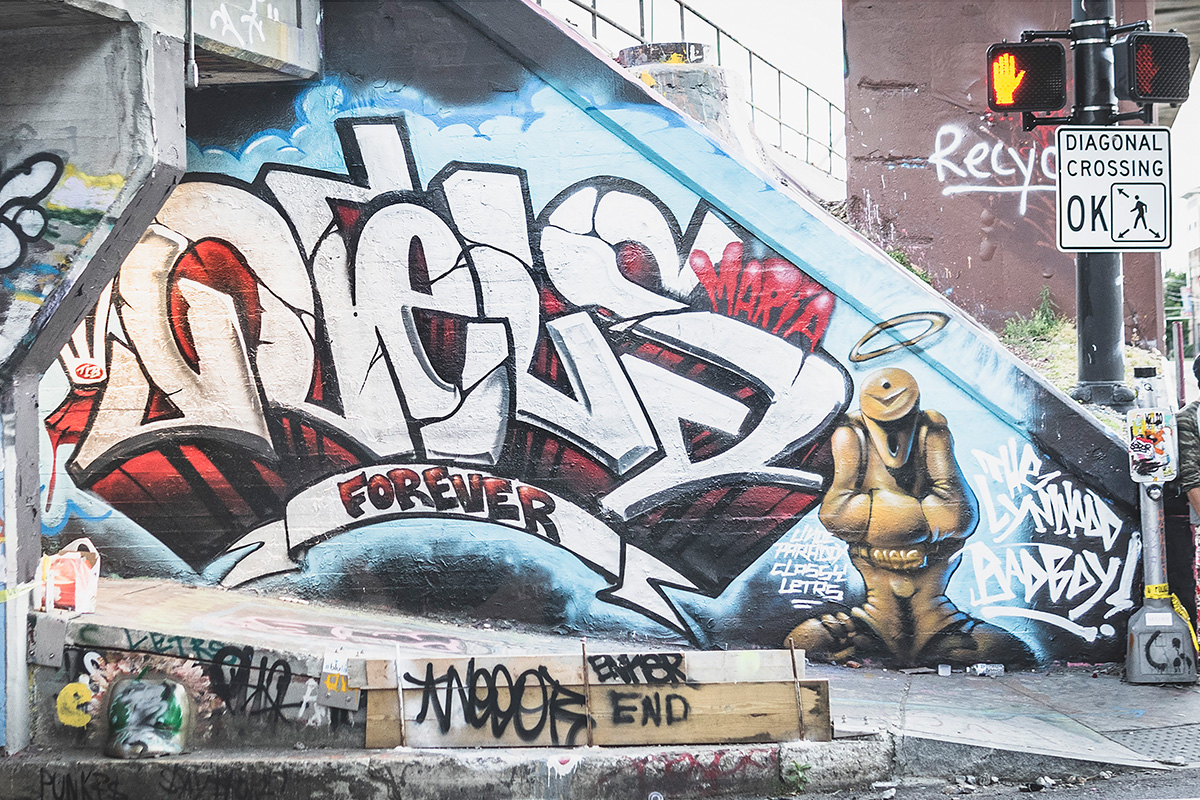The photograph, in landscape orientation, captures a bustling city street centered around a vividly painted graffiti mural on the side of a staircase. The staircase leads up to a bridge on the left side of the image, and there is a ramp at the front, seemingly intended for handicap access. The mural, notable for its bold letters and layered artwork, features the name "Maria" in white letters with a red drop shadow, accompanied by a banner that reads "Forever." A figure with a halo, an alien-like creature in a space suit, and additional intricate designs add to the vividness of the graffiti. Below the mural, several boards have been tagged with black spray paint. To the right of the staircase, there is a crosswalk and a traffic sign displaying a flashing yellow caution signal. The setting is further detailed with decaying buildings in the background and a slightly dirty sidewalk in the foreground. Overall, the image epitomizes an urban environment rich in street art, characterized by photographic representational realism.